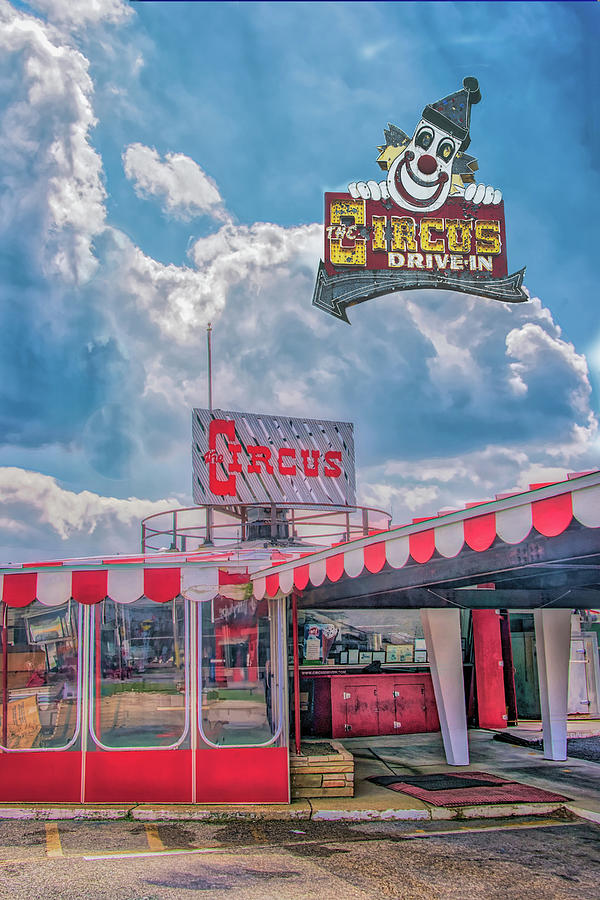The photograph captures a vintage circus-themed drive-in restaurant, its appearance marked by a sense of abandonment and dilapidation. The sky is a blend of blue and cloudy, with dark, ominous clouds forming. In the foreground lies a vacant parking lot that leads up to the building. The building itself features a distinctive circus theme, adorned with a red and white alternating banner that scallops along its roofline. Prominently, a sign that appears to be floating in mid-air—despite likely being mounted on an unseen post—shows a large white neon clown face holding an arrow, reading "Circus Drive-In." Another red sign on top of the building simply says "Circus." The windows and counters hint at its former function as a place where cars would pull up to be served, capturing a nostalgic element of past roadside Americana.